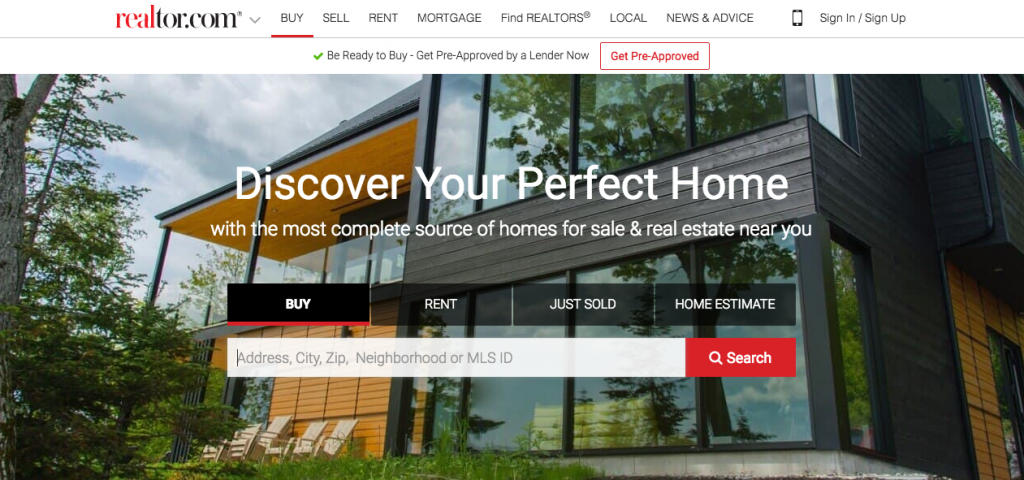The image features a screenshot from Realtor.com. The "Real" and "Realtor" are highlighted in red, while "Ter.com" is in black. At the top navigation bar, a gray down arrow appears with several black submenu labels: "Buy" (underlined in red), "Sell," "Rent," "Mortgage," "Find Realtors," "Local News," and "Advice." On the far right, a black cell phone icon accompanies the option "Sign In/Sign Up." Below this, a gray line divides the header from the advertisement below. A green check mark next to the text reads, "Be ready to buy; get pre-approved by a lender now," beside a red box with the text "Get Pre-Approved."

Beneath the header, there's an image of a sleek, modern home with a mix of orange and black siding, massive glass windows, and surrounding greenery, including trees and lawn chairs. Clouds dot the sky above. Superimposed on the image in white text is the message: "Design your perfect home with the most complete source of homes for sale and real estate near you."

Continuing down, the site features black and white navigational boxes labeled: "Buy" (underlined in red), "Rent," "Just Sold," and "Home Estimate." Below these options, a prominent white search box invites users to enter an "Address, City, Zip, Neighborhood, or MLS ID," followed by a red and white search button with a white magnifying glass icon. Reflections of trees and sky are visible in the house's large windows, contributing to the clear and visually accessible design of the site.